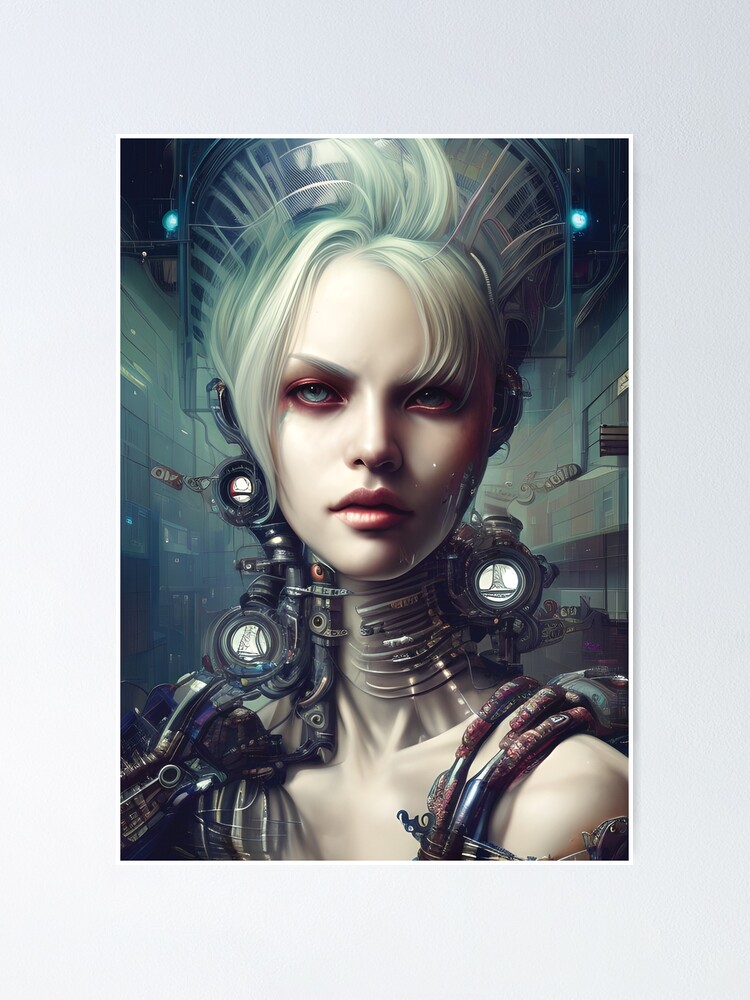The image depicts a captivating, digitally rendered portrait of a futuristic woman in her mid to late 20s, characterized by her striking, refined features, full lips, and crystal blue eyes. Her blonde hair, styled in a punk fashion with tufts swept over her forehead and sticking up towards the back, drapes slightly over her face, adding an air of mystery.

She is adorned with an elaborate mechanical apparatus that wraps around her neck and shoulders, composed of dark metal structures, small round lenses, and cables that hint at some advanced functionality or purpose. The device spans over her left shoulder and further extends over her right, with additional semi-organic metallic components that could be sensors or other intricate devices. These elements contribute to her potential identity as a cyborg, though it remains ambiguous.

The backdrop of the image suggests an industrial or futuristic setting, possibly the interior of a technological facility, with greenish-blue and dark gray hues, and dim lighting that highlights the mechanical ambiance. A soft light from the left side of the image casts a gentle glow across her face, contrasting with the shadow on her right side, which adds depth and enhances the dramatic effect of the scene.